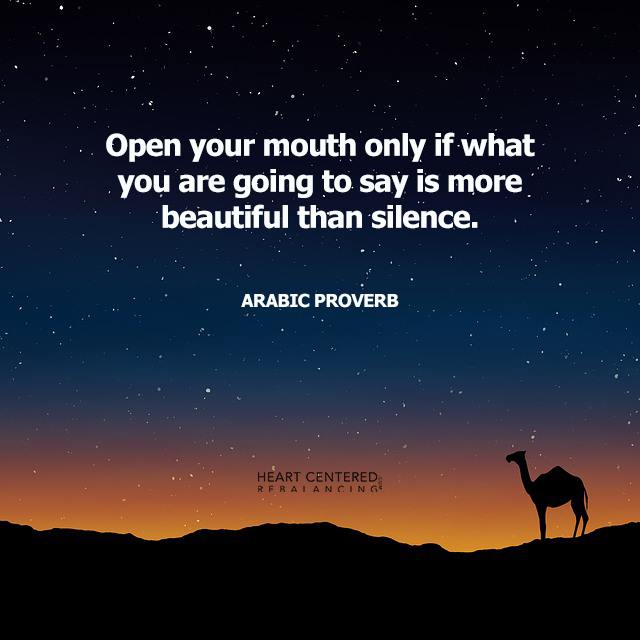This tall, rectangular ad features a striking digital artwork and an evocative Arabic proverb. The foreground presents a simulated silhouette of a single-humped camel with a tail, standing on a hilly surface on the right side, gazing left. The intricate background transitions smoothly from a deep orange band of a sunset at the bottom through lighter shades of blue, culminating in a dark blue to black night sky sprinkled with stars. Bold white text centered at the top of the image proclaims, "Open your mouth only if what you are going to say is more beautiful than silence," followed by the attribution "Arabic Proverb" in all capital letters. Just left of the camel, the phrase "HEART-CENTERED REBALANCING" is subtly positioned, completing the sophisticated and calming aesthetic of the ad.